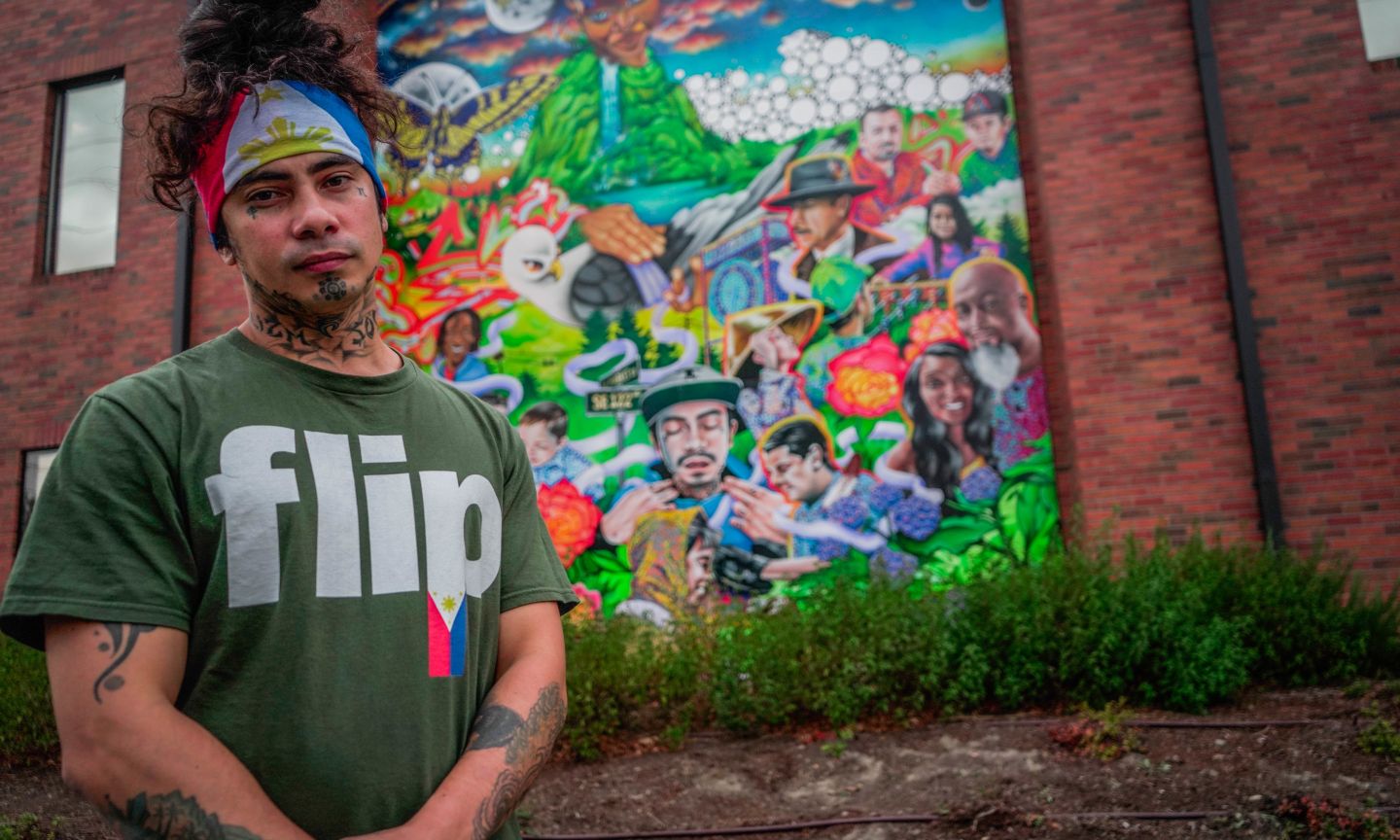The image depicts a vibrant outdoor mural on the side of a brick building, illustrating an array of bright colors and intricate designs, including various people interacting, trees, flowers, a bird, and some terrain. A prominent figure in the mural is a man with a mustache. In front of this artwork stands a young, brown-skinned man who appears to be in his 20s. He has short to medium curly hair held up by a thick bandana, which features the colors of the Filipino flag. His face, neck, and arms are covered in tattoos, suggesting possible gang affiliations. He wears a green t-shirt with the word "Flip" on it, where the 'P' has an interlinking red and blue color design, evocative of the Filipino flag. The scene includes boxwood hedges neatly trimmed in front of the wall, adding to the lush and engaging outdoor setting. The man's stance and expression imply he could be the artist behind the mural, though this is not certain.